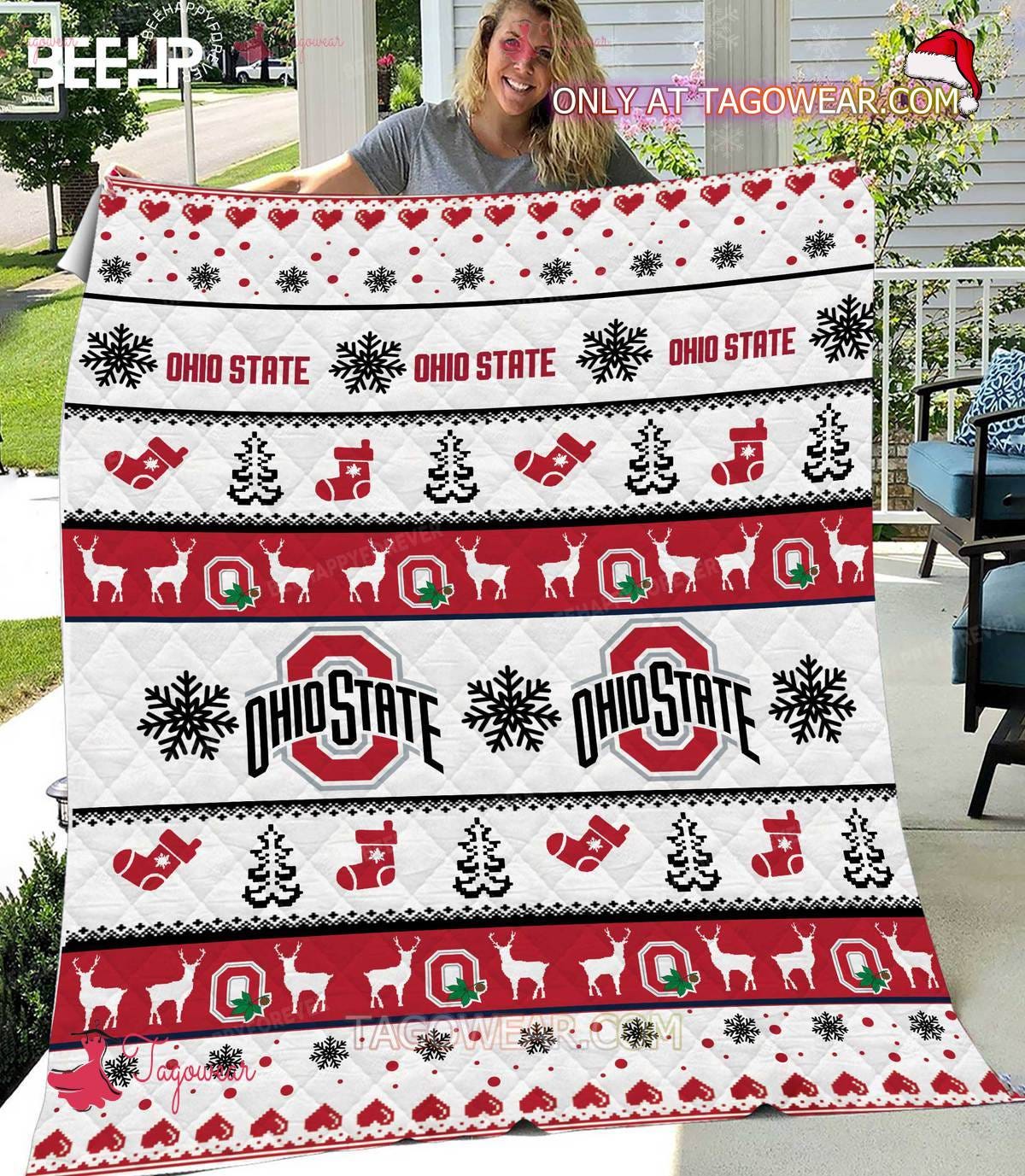This photograph captures a woman standing on her porch, holding up a festive quilt prominently themed around Ohio State and Christmas. The quilt’s bold design includes striking colors of red, white, black, and green, adorned with various holiday motifs such as Christmas trees, stockings, reindeer, hearts, and Santa Claus hats. Notably, black snowflakes are woven throughout the quilt alongside multiple instances of “Ohio State,” including sections featuring the Ohio State logo with a buckeye leaf. 

At the top edge of the quilt, the text "only at tygoware.com" is visible, although partially obscured, and to the top left, the letters "G-E-E-H-P" can be made out. The woman holding the quilt has long blonde hair, is smiling, and is dressed in a gray sweatshirt. She's posed with outstretched arms on her porch, which has a couple of chairs and a railing visible, with a sunny, summertime neighborhood backdrop including the lawn, street, and a neighboring house wall.